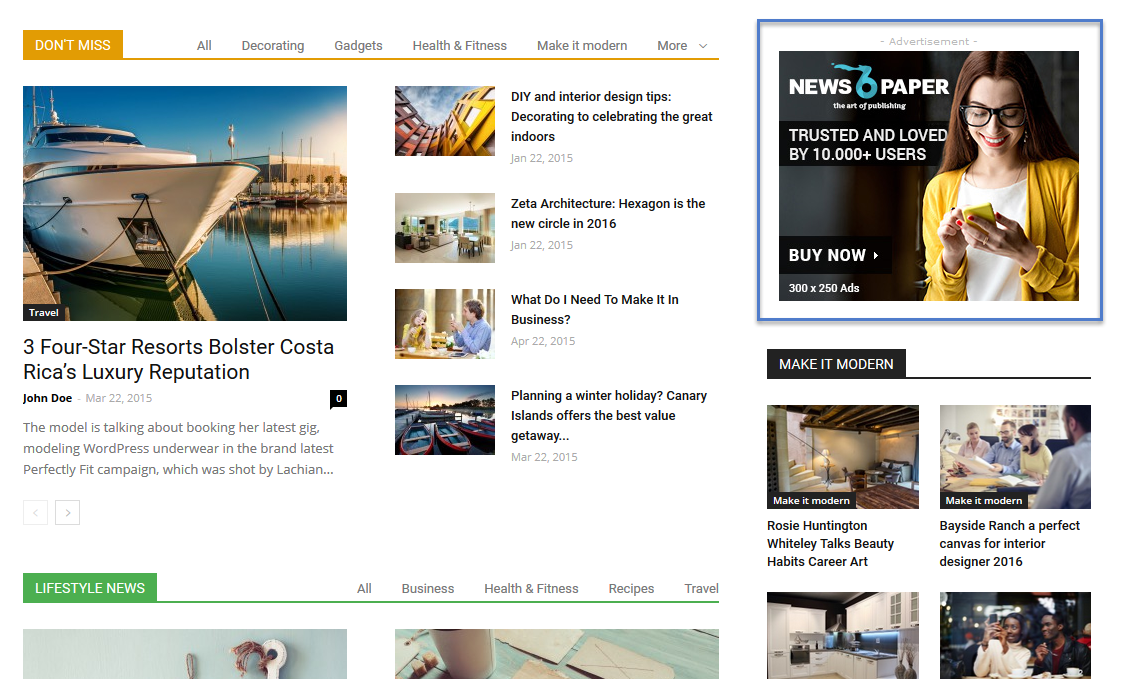A screenshot with a white background features various elements arranged in an organized layout. At the top of the image, within an orange rectangle, white text reads "Don't Miss." The screenshot showcases a variety of topics including decorating gadgets, health and fitness, modern designs, and more. 

Central to the screenshot is an image of a serene boat floating on the water, with a distant building on the horizon, suggesting a tranquil travel locale. Below the image, three luxury four-star resorts in Costa Rica are highlighted, emphasizing the country's growing reputation in luxury travel. The accompanying text, attributed to John Doe, is dated March 22, 2015 and notes that a model is discussing her latest booking for a gig. This gig pertains to a campaign for ModelingWordPress (with capitalization as "ModelingWordPress"), specifically for an underwear brand's "Latest Perfectly Fit" campaign, reportedly shot by someone named LACHIN.

Navigation arrows on the left and right sides of the image indicate additional content available for viewing. 

The right side of the screenshot lists several articles, including:

1. DIY and Interior Design Tips: Decorating to Celebrate Indoors (January 22, 2015)
2. Zeta Architecture: Hexagon is the New Circle in 2016 (January 22, 2015)
3. What Do I Need to Make it in Business? (April 22, 2015)
4. Planning a Winter Holiday: Canary Islands Offers the Best Value Getaway... 

These articles offer a broad range of topics from interior design to travel tips, catering to varied interests.